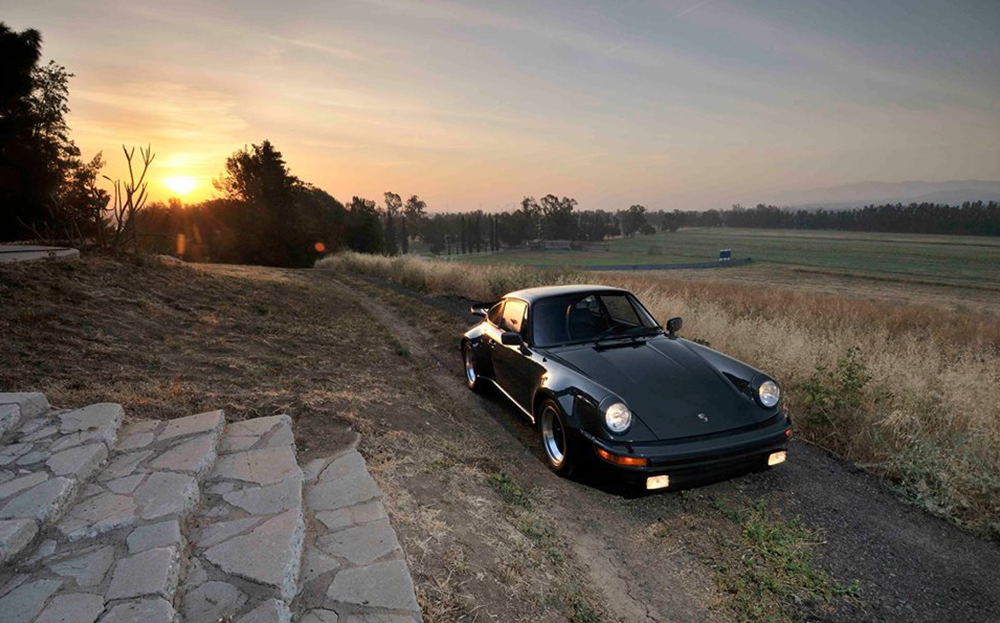In this horizontal, color landscape photograph taken outdoors at dusk, a sleek black Porsche sports car, with its running lights on, sits parked on an unpaved dirt road, facing the camera. The surrounding area is expansive, with vast open fields extending to both sides of the road and a distant tree line illuminated by the golden glow of the setting sun. On the left side of the image, a series of wide stone stairs ascend towards an unseen destination, while on the right, the fields stretch out into the distance. The car appears unoccupied, enhancing the serene, twilight atmosphere of the scene.